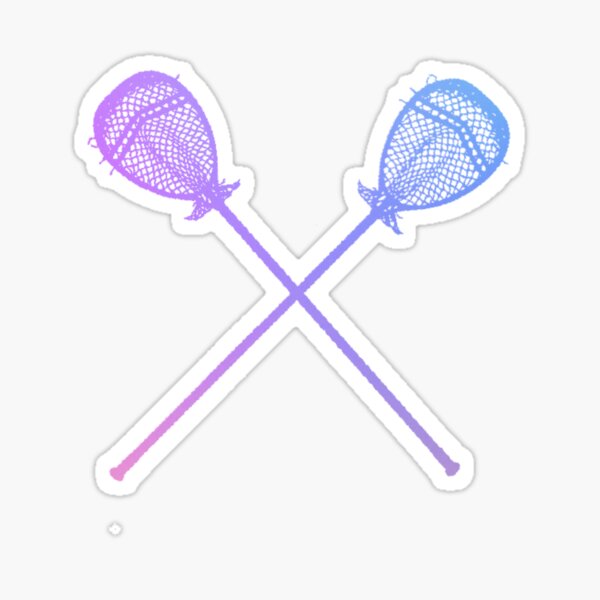The image depicts an emblem featuring two crossed lacrosse sticks on an off-white background with a thin gray outline. The sticks intersect diagonally, one originating from the lower right corner and extending to the upper left, while the other starts at the lower left and extends to the upper right. The lacrosse stick on the left side has a gradient colored handle, starting purple at the base and transitioning to blue at the net. The stick on the right is purple with a distinct net at the top. The elegant design and color transition suggest a modern and stylized representation of lacrosse equipment, featuring elongated handles and oval-shaped nets. The overall aesthetic combines the traditional elements of lacrosse with contemporary design elements, making the emblem visually striking.